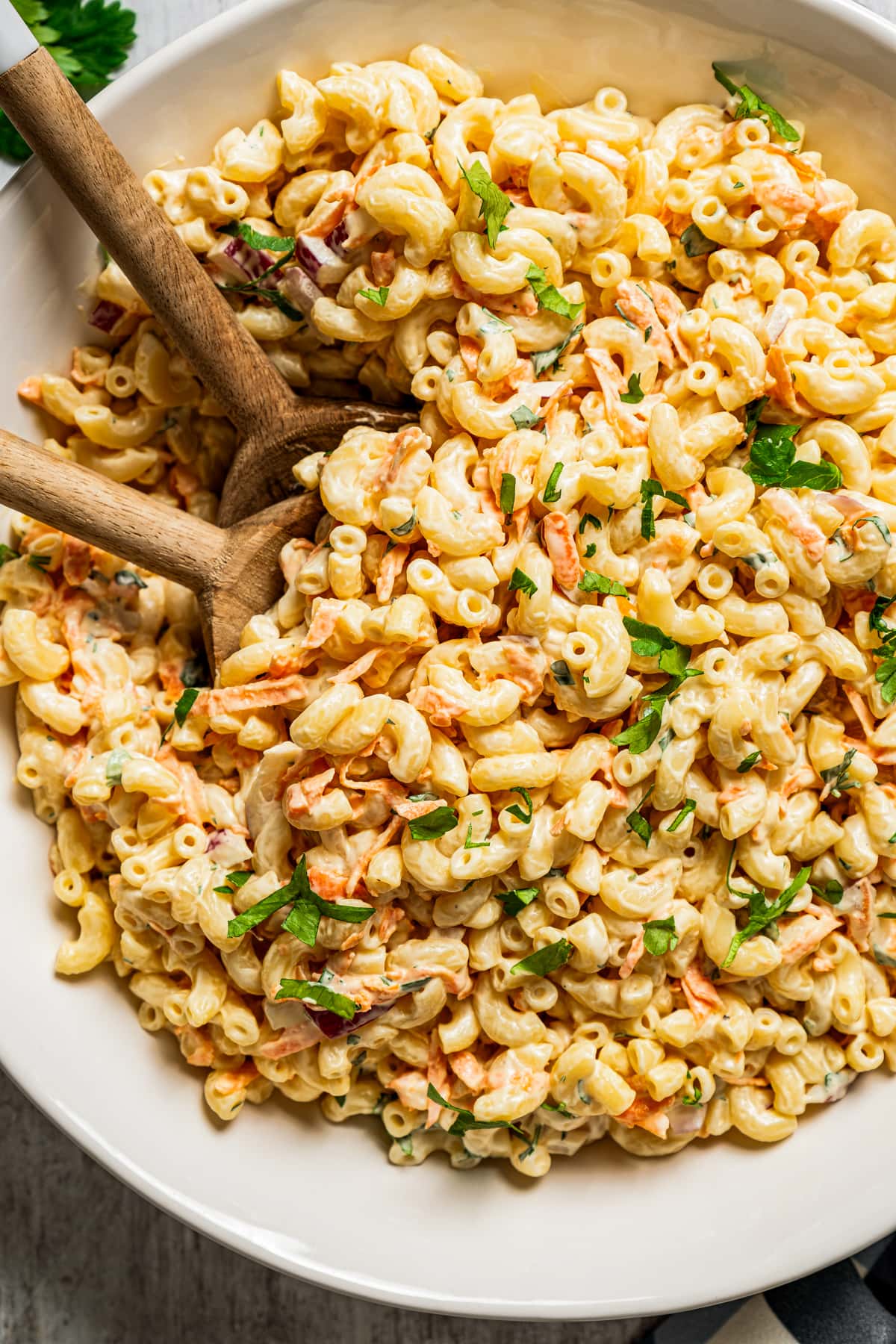This detailed close-up photograph showcases a large, round white ceramic bowl of pasta, viewed from a top-down perspective. The pasta, consisting primarily of elbow noodles, is generously coated in a light orange, cheesy sauce, which gives it a creamy appearance. Scattered throughout the dish are bits of green herbs, likely parsley and basil, adding a fresh touch. The pasta also includes small chunks of meat, possibly chicken or bacon, and some orange-tinted ingredients that may resemble carrots. 

Two roughly crafted wooden spoons are partially submerged in the pasta, one with a dark brown handle and bowl, the other with a lighter brown handle and bowl, both inserted into the bowl from the top left corner and converging towards the center. The entire composition sits on a light-colored wooden surface, with a visible parsley leaf at the very top left corner outside the bowl, adding a final garnish to this visually appealing dish.